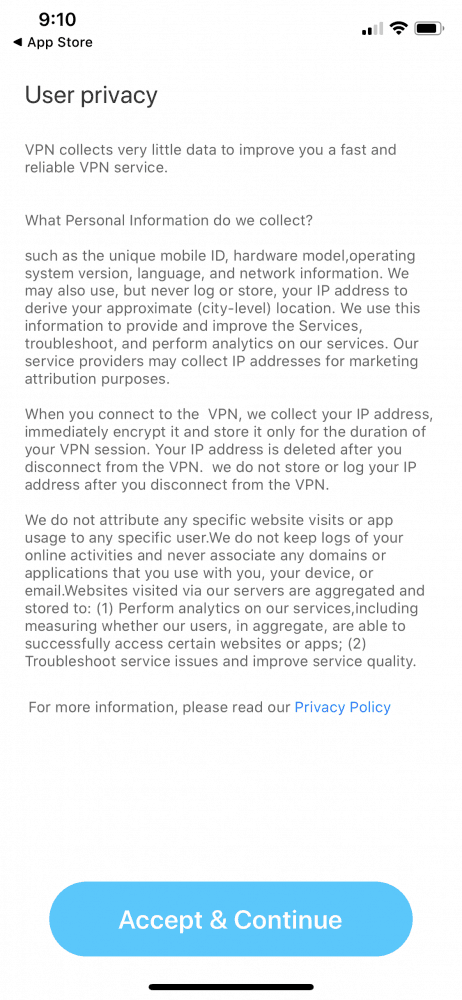A screenshot taken from a mobile device displays the App Store interface. 

- **Top Bar:**
  - *Time:* 9:10 in the top left corner.
  - *Indicators:* Wi-Fi signal strength, cellular signal strength, and battery icons on the top right.

- **Header:**
  - *Navigation:* A back arrow followed by the text "App Store."

- **Main Content:**
  - *Title:* "User Privacy"
  - *Text:* The screen outlines the VPN service's data collection practices:
    - **Data Collected:** Unique mobile ID, hardware model, operating system version, language, and network information.
    - **IP Address Usage:** IP addresses are collected, encrypted, and stored only for the duration of the VPN session, and deleted upon disconnection.
    - **Usage Assurance:** No specific website visits or app usage are linked to any individual user. No logs of online activities are maintained.
    - **Purpose:** Data is aggregated to perform service analytics, troubleshoot issues, and improve service quality.

- **Footer:**
  - *Action Button:* A blue button labeled "Accept and Continue."